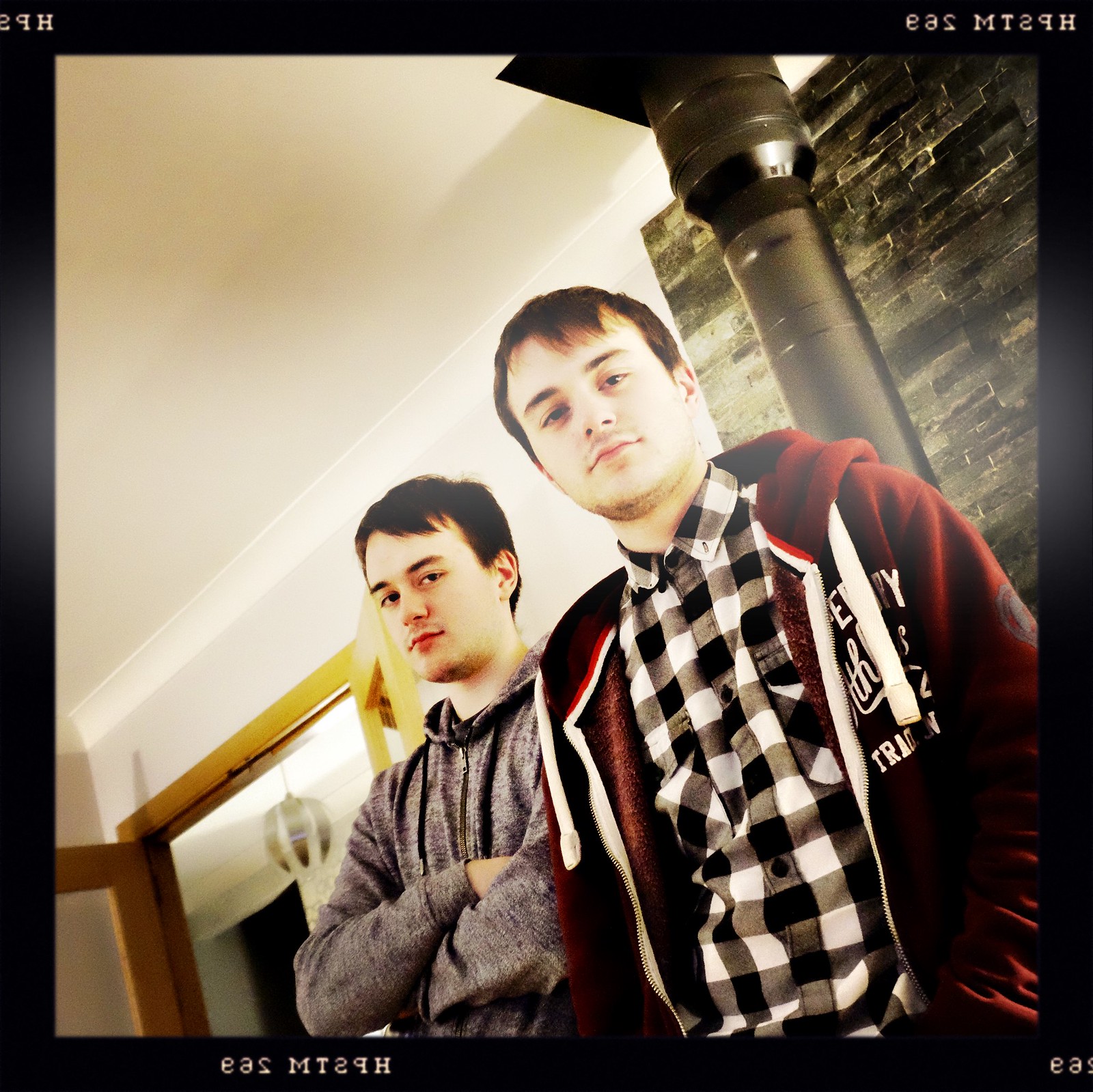The photograph features two teenage boys, both of whom are Caucasian and looking directly at the camera. The image is bordered by a black frame with random, and sometimes nonsensical, characters, including one that resembles a backwards number two. The boy on the right is dressed in a black and white checkered flannel shirt with a red (or maroon) hoodie over it, distinguished by white strings and a white zipper. His hair is short and brown, and he stands with his hands positioned near his waist, where they might be in his pockets, although this area transitions into darkness. 

The boy to his left, slightly behind the first boy’s shoulder but still prominently visible, has light brown hair and wears a gray hoodie. His arms are crossed over his chest. The background features a mix of architectural elements: to the right, there's a structure that appears to be a stone fireplace, while elsewhere, white walls are accented with light wood trim. A doorway and a possible chrome pillar in front of a brick facade are also partially visible, suggesting the scene is set inside a room.